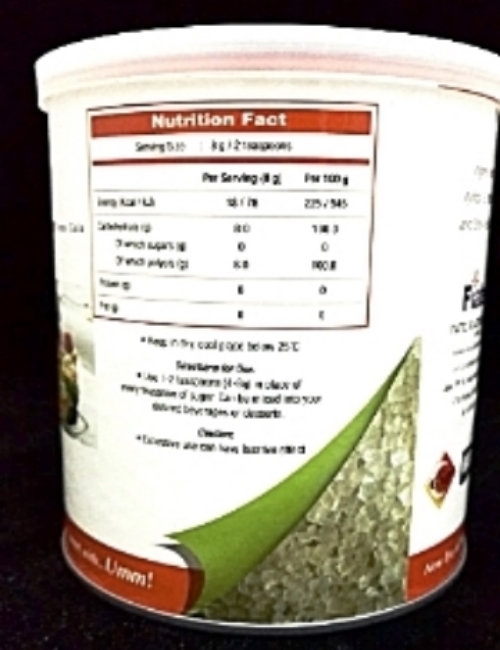A slightly blurred photograph showcases the backside of a white plastic container, likely for ice cream or yogurt. The container features a red band at the bottom, with barely legible white lettering on it. The middle section of the container appears to have a portion pulled up, revealing a green area beneath. Adjacent to the green section on the right is a brownish-gray area that resembles dirt or rock. The rest of the container is predominantly white, with standard nutritional information printed on it. The nutrition facts are displayed in a white box with a red border and black text, although the text is largely out of focus and unreadable. To the right, some logos are present but similarly blurred and illegible. The background of the image is solid black, emphasizing the container's features despite the overall lack of clarity.